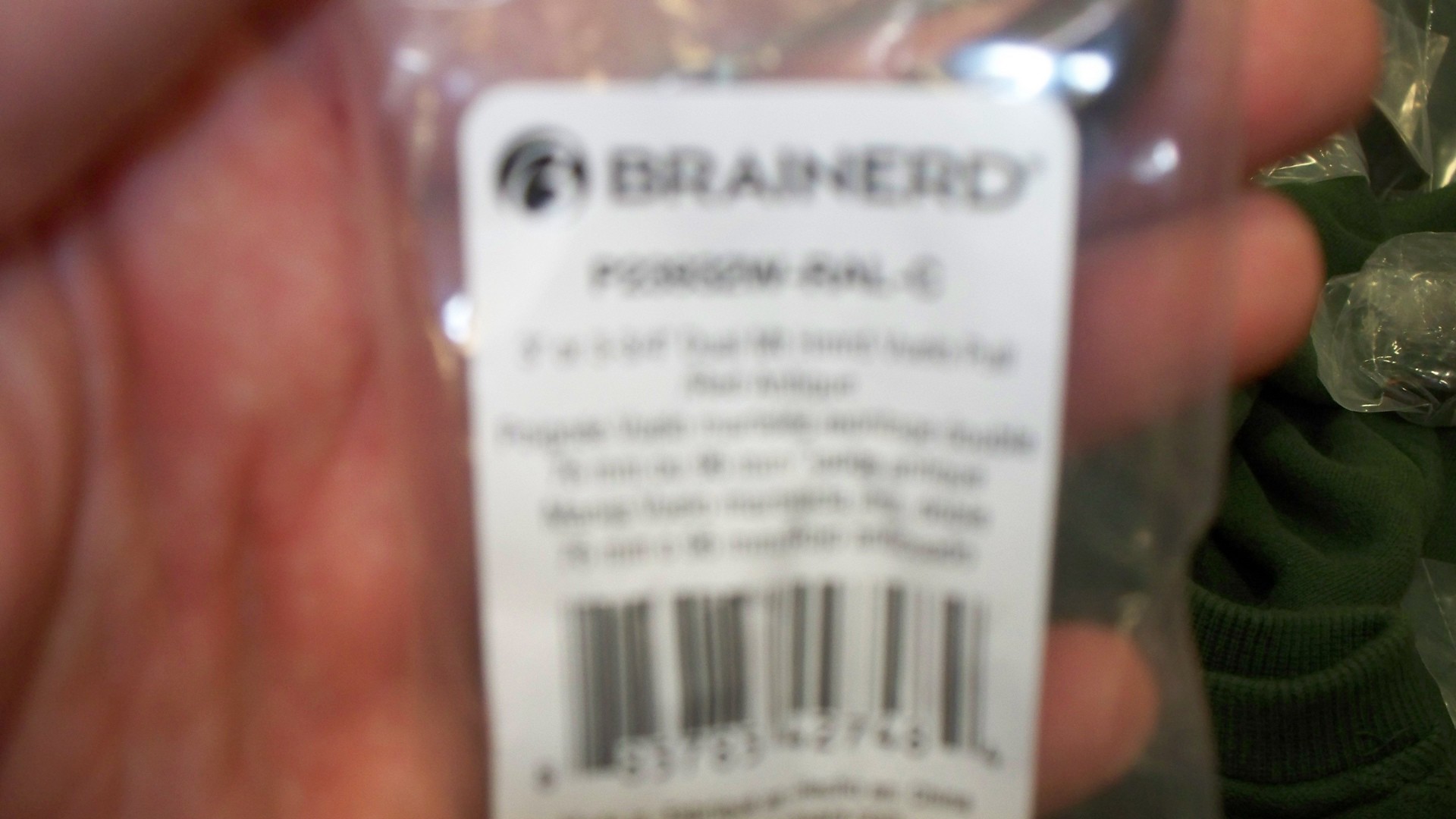This image depicts a blurry photograph of a product label, primarily focused on a barcode. The label is almost indecipherable due to camera movement during the capture. At the top of the label, faint and unclear text appears to spell "Brain Nerd," "Bread Nerd," "Bradge Nerd," or a similar variation. The product is held by a person with a fair complexion, using their left hand.